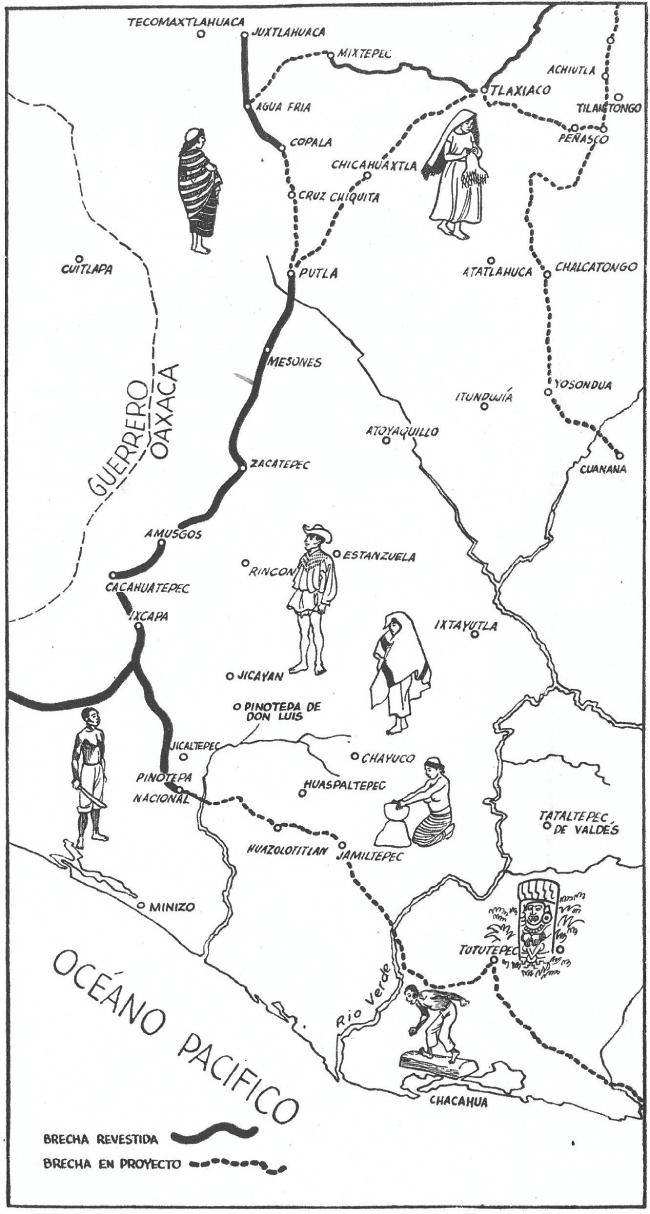This black and white line drawing map depicts a portion of southern Mexico, focusing primarily on the areas bordering the Pacific Ocean, labeled as "Oceano Pacifico" in Spanish at the lower left corner. The map showcases various towns and cities marked by small dots, rivers such as Rio Verde, roads, and potentially areas of construction. Notably, there is a distinction made by borders between the states of Guerrero and Oaxaca delineated by a dotted line in the upper left.

Scattered across the map are intricate drawings of people in traditional attire, indicative of the local culture. These include a shirtless man with a machete and rolled-up linen pants, a man seeming to balance on a log, possibly depicting a traditional activity, and a woman sculpting pottery. Additionally, there are women dressed in attire resembling nuns with shawls and ankle-length dresses, and a man in a cowboy hat with a poncho. Unique lines represent different types of routes: dark lines signify "Breca Revistida" (paved roads) and dotted lines "Breca in Proyecto" (planned routes), as indicated by the key at the bottom left.

Overall, the map is a detailed illustration highlighting not only the geographic features and urban planning of southern Mexico but also giving a glimpse into the cultural elements through its artistic sketches.